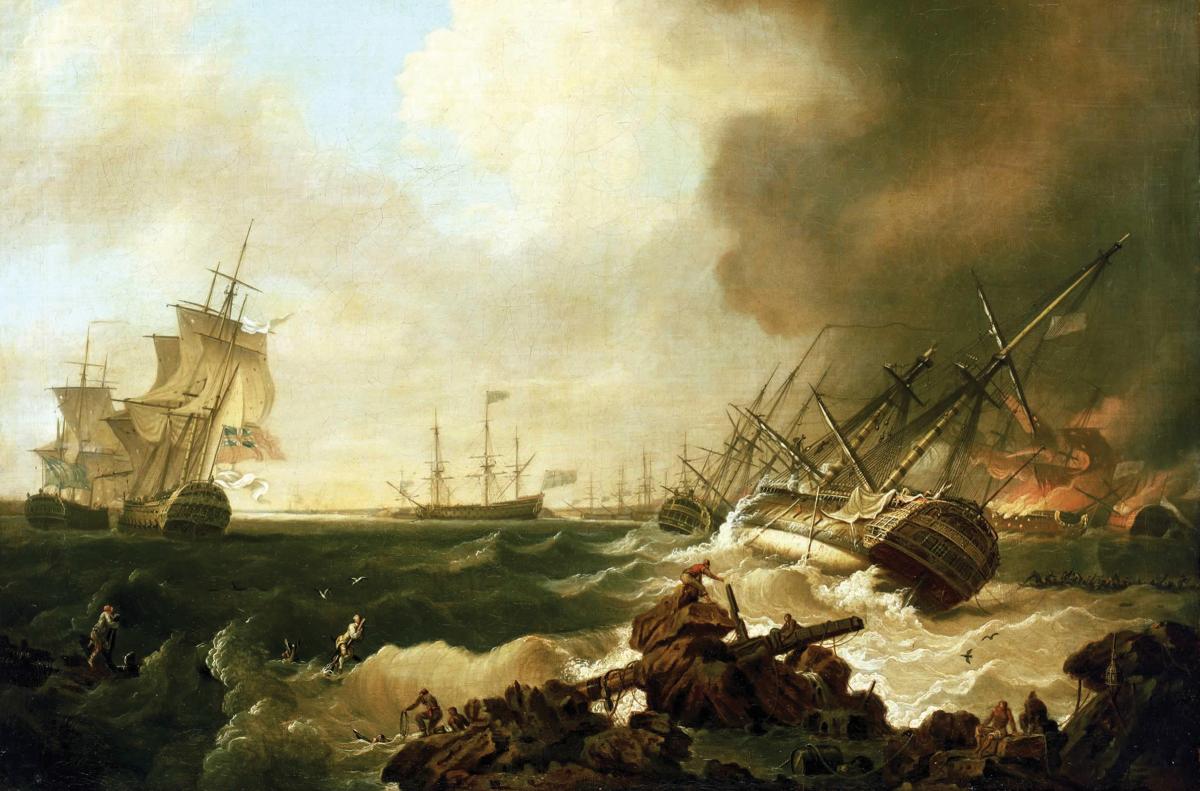The image is a highly detailed landscape, likely an oil painting or a very realistic digital creation, depicting a tumultuous sea battle involving colonial-era ships. The ocean's dark, bluish-gray waves are punctuated by white caps, illustrating the rough waters that toss the ships. A dramatic sky stretches above, divided between the clear blue on the left and storm-filled clouds on the right, interspersed with brown and white smoke plumes from fires.

There are six ships in total, sailing with numerous masts and billowing sails. On the left, the front ship prominently flies a British flag. Two ships are in the process of capsizing, nearly overturned by the ferocious waves. In the background, another ship is ablaze, sending thick smoke into the sky. Additional flags can be seen fluttering on distant ships.

In the foreground, people are seen on the shore, appearing to be either survivors or rescuers. Some are navigating through debris from wrecked ships, trying to reach the safety of the land. The painting captures the chaotic scene with meticulous detail—the fierce ocean, the embattled ships, the engulfing flames, and the anxious figures on the shore—all contributing to an evocative portrayal of maritime conflict.